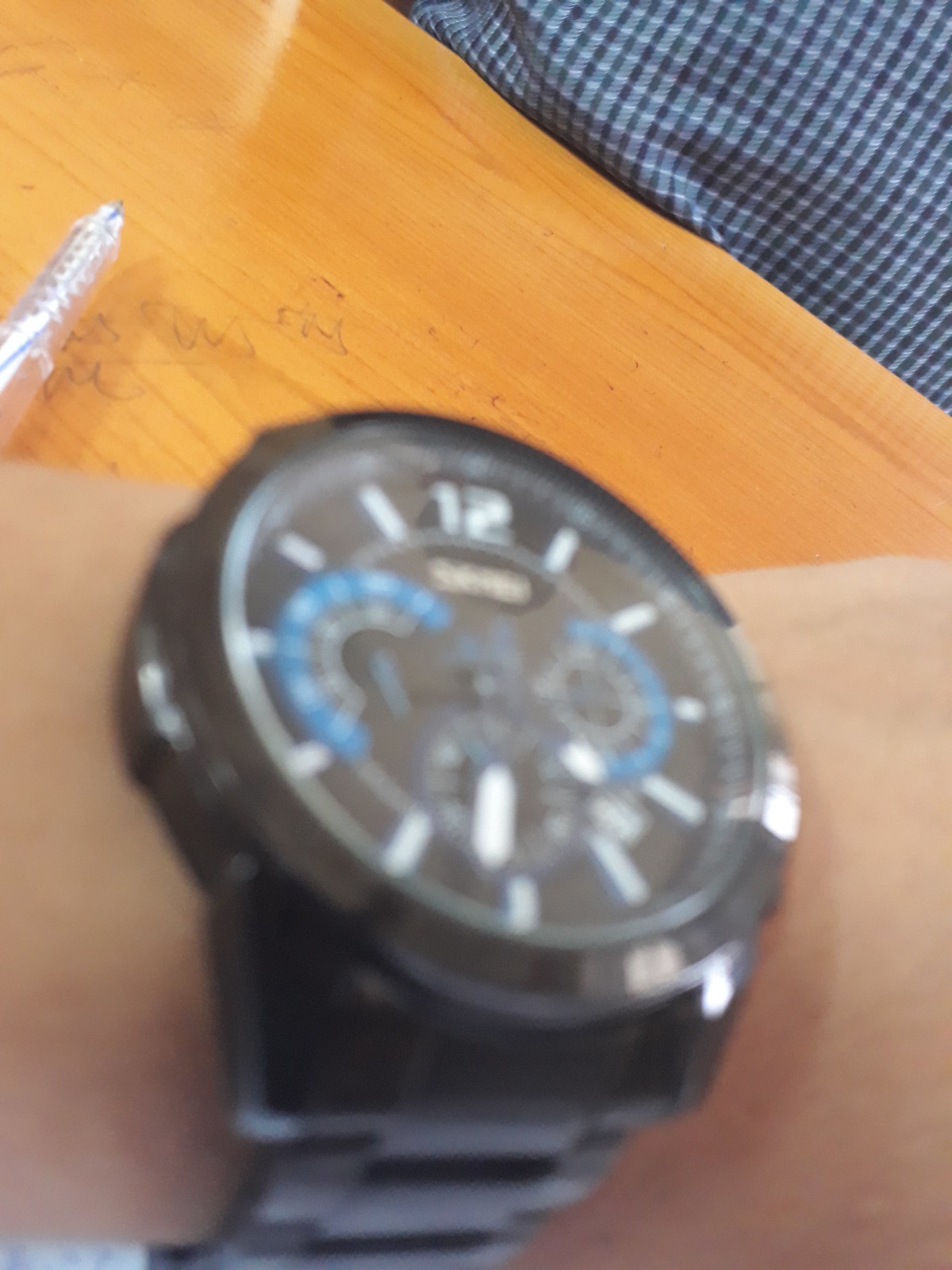This photograph captures a wristwatch on a person's wrist, viewed from above. The watch features a black band, a black face, and a black encircling ring. The number "12" is clearly displayed at the top in white, while the remaining numbers are represented by silver notches. Two blue half-circle designs are situated within the center of the watch face. The hands of the clock appear to be black with white tips. The wristwatch has a thick, sturdy, and masculine appearance, although many details of the watch are blurred due to the camera's focus on the background instead of the watch.

The background is the upper half of the photograph, showing a light golden-colored wooden table marked with faint, washed-out graffiti or scribbles. A clear plastic ink pen lies on the upper left corner of the table. In the upper right corner, a blue checkered shirt is visible, pressed up against the table's edge. The person's arm and part of their hand can also be seen, further emphasizing the casual setting of the shot.